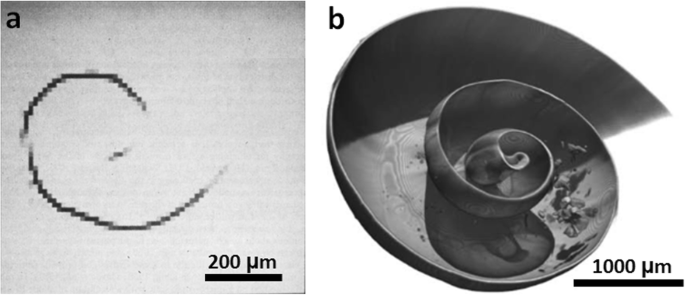The composite image comprises two square-shaped photos positioned side by side, with the left showcasing a 2D drawing and the right a 3D model. The left image illustrates a simple, curved black line over a gray background, resembling the tracing of a spiral. In the top left corner, the letter "A" is visible, while the bottom right corner features a scale marked "200 µm." The right image presents a detailed 3D drawing, depicting a spiral-shaped object that resembles a shell, possibly made from ceramic or clay, set against a white background. This image is marked with the letter "B" in the top left corner and a scale reading "1000 µm" in the bottom right. Both images are rendered in grayscale tones, including dark gray, black, and off-white, and are likely digitally created to illustrate the differing scales and dimensions of the depicted objects.